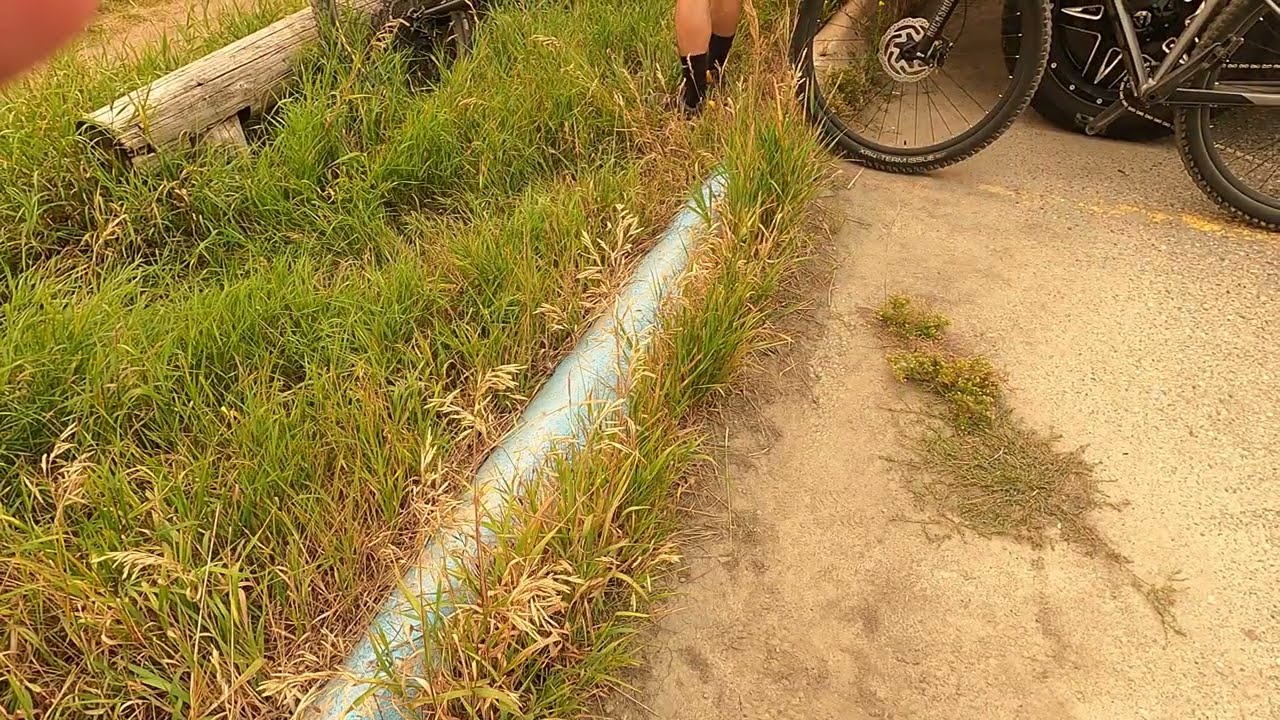The image depicts an overgrown parking lot with a dirt-covered surface, interspersed with patches of grass and vegetation breaking through the pavement. Prominently, a black and gray bicycle with rugged tires is parked along a faded yellow parking spot line. To the left, an area dense with greenery features an old, dried-out wooden log and a man wearing brown shoes and black socks standing at the upper edge of the image. The top left corner is slightly obscured by a finger, presumably from the person taking the photo. Behind the bicycle, a car with black tires and black and silver rims is partially visible. Additionally, a silver-colored pole is seen on the curb. The entire scene has a distinct orange-yellow hue, possibly due to the lighting or camera settings, enhancing the rustic, almost desert-like atmosphere.